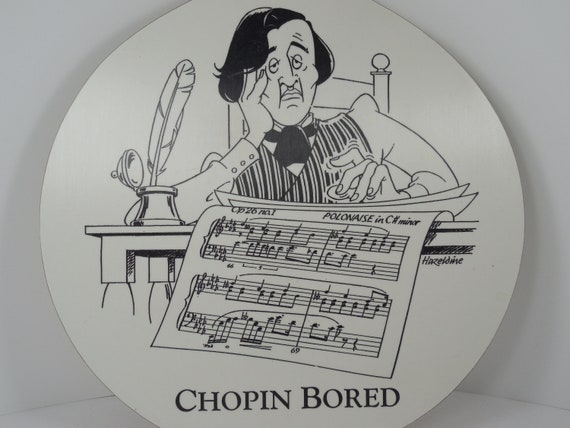The image is a photograph of a circular decorative object, likely a plate or an art piece, resting on a white surface against two white walls. The design features a black and white cartoon-esque illustration that parodies famed composer Frédéric Chopin in a humorous, bored state. The artwork depicts Chopin sitting at a desk, strumming his left fingers on the tabletop while his right hand props up his face, conveying a sense of ennui. He's adorned in a string tie, a striped vest, and a white shirt. On the desk, there is an inkwell with a feather quill, and a sheet of music titled "Polonaise in C minor" appears to be sliding off towards the viewer, with musical notes and staffs visible. The illustration is captioned with a pun, "Chopin Bored," playing on the words 'chopping board' and the composer's name, adding a whimsical touch to the piece.